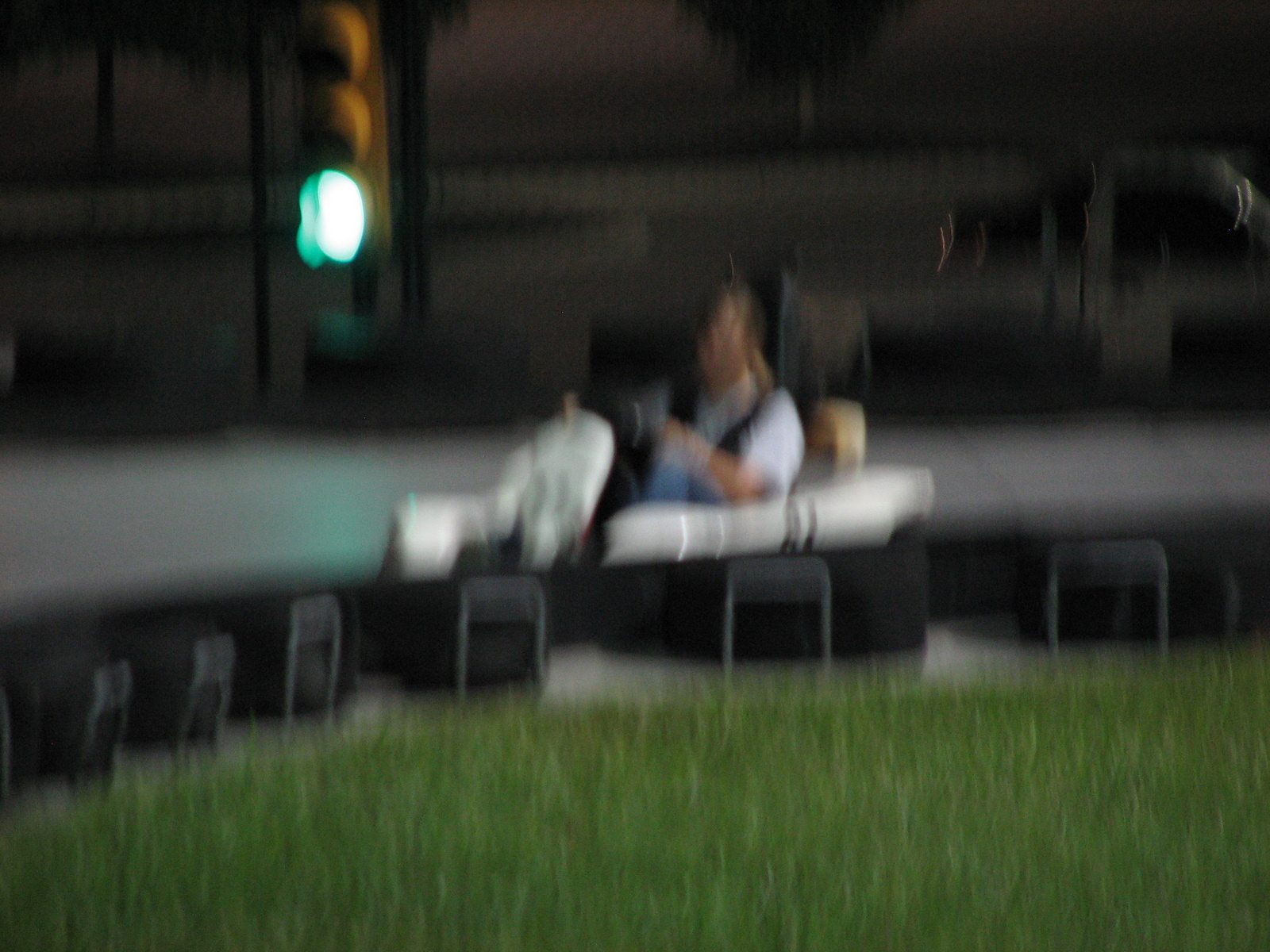In this somewhat blurry image, a woman with a ponytail is captured either standing or sitting near a white pipe, seemingly engaged in a task. She wears a white blouse paired with a black vest. Her left arm is positioned close to the white pipe, and both hands are actively working on another white object that appears to be a part of the pipe. The environment features a mix of black boxes and grass, creating a puzzling scene as her position appears to be at the same level as a green traffic light nearby. This unusual alignment of elements adds to the intrigue of the image.